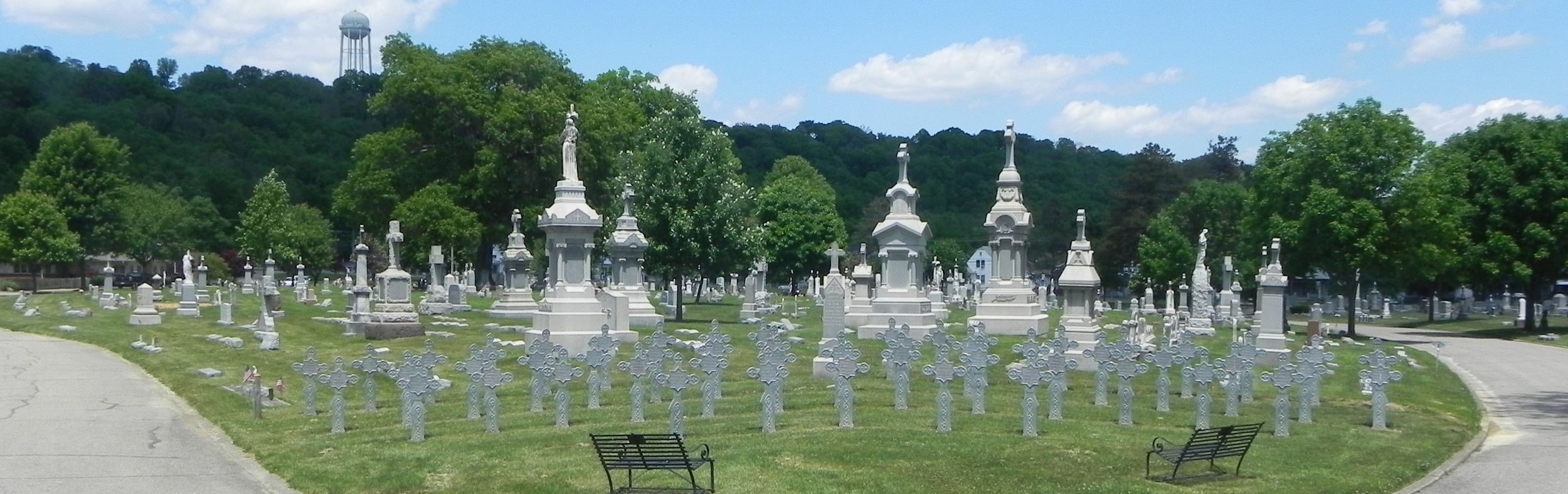The photograph is a long vertical rectangle capturing a neatly arranged portion of a cemetery. The image showcases two small roads framing the cemetery, one curving from the bottom right corner and the other entering from the left side. The cemetery includes orderly rows of approximately 30 identical ornate gray crosses, arranged in about three rows at the foreground. In the middle ground, there are larger, tall monument-style markers and some smaller stones to the left. Two black benches are positioned at the front of the graveyard plot.

Surrounding the cemetery are lush green trees, with some lining the distant road seen on the right. The background reveals a slight hill also covered with trees, and a prominent white water tower is visible in the upper left part of the photograph, set against a sky with scattered clouds.